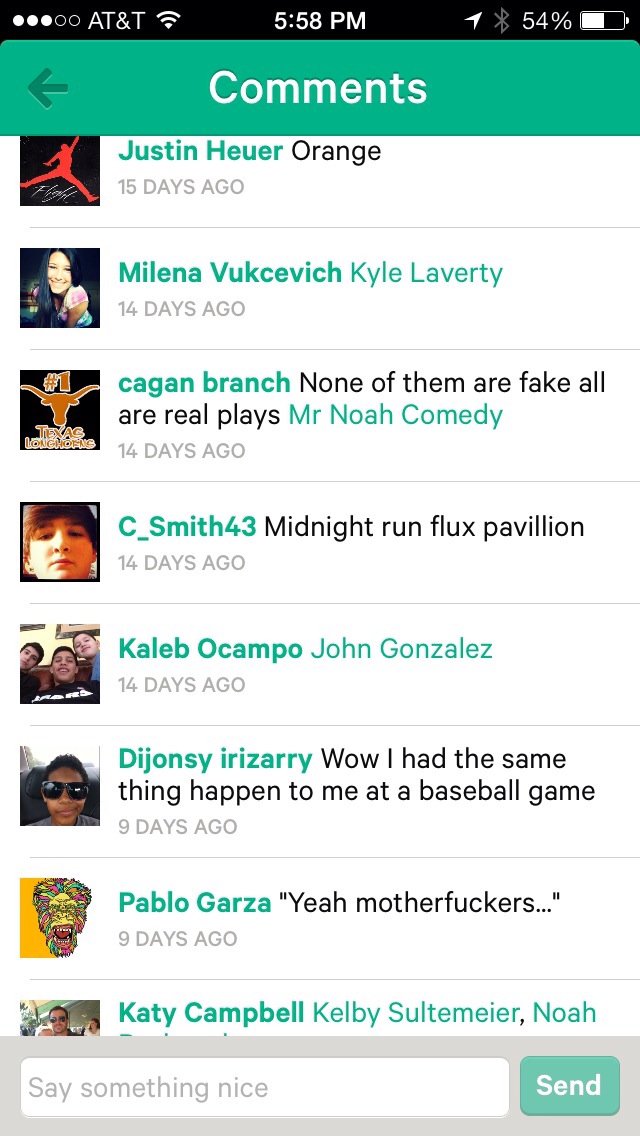This image is a vertical rectangular screenshot of a mobile phone displaying the comment section of a website or app. At the top, a standard black horizontal status bar shows AT&T service with three out of five signal bars, the Wi-Fi icon, the time (5:50 p.m.), and a 54% battery level. To the right of the time, there are icons for messages, Bluetooth, and the battery status.

Below the status bar is a large aqua-colored horizontal strip with white text that reads "Comments" in the center and a back arrow on the left. The comment section contains eight comments, each identified by the user's name in aqua color, their profile picture on the left, and their comment in black text. Additionally, the timestamp of each comment is noted below the user's name.

The comments and their respective users are as follows:
1. Justin Heuer commented "orange" 15 days ago.
2. Milena Vesuvik mentioned "Kyle Laverte" 10 days ago.
3. Kagan Branch stated, "none of them are fake, all are real plays" Mr. Noah comedy, 10 days ago.
4. C. Smith 43 wrote "midnight run flux pavilion" 14 days ago.
5. Caleb Ocampo remarked "John Gonzalez" 14 days ago.
6. Djonze Irizarry shared, "Wow, I had the same thing happen to me at a baseball game" 9 days ago.
7. Pablo Garza quoted, "yeah, motherfuckers..." 9 days ago.
8. Katie Campbell lastly chimed in with a comment not shown in full detail.

At the bottom of the comment section is a horizontal gray strip with a blank white text box that says "Say something nice," accompanied by a green send button in the right-hand corner, ready for new input.